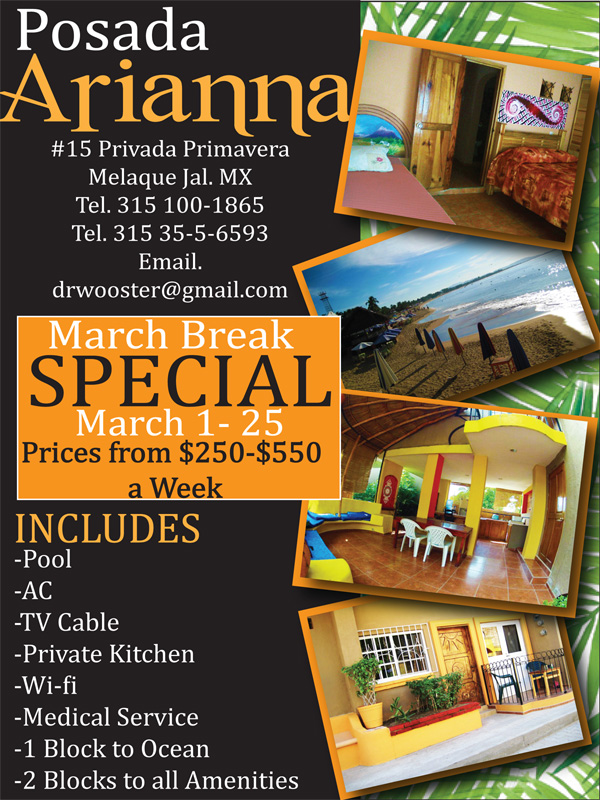This image features an advertisement for hotel rooms at Posada Ariana, showcasing a vibrant, Mexican-Spanish style atmosphere. The ad is divided into two sections: the left side is dark gray with white and orange lettering, while the right side features four staggered, colorful photographs.

On the left, the ad provides essential details in various colors: the hotel name, Posada Ariana, is highlighted at the top, followed by the address (No. 15 Privada Primavera, Malik, QJ, LMX), two telephone numbers, and an email contact. Below this, an orange rectangular section announces a "March Break Special" from March 1st to 25th, with prices ranging from $250 to $550 per week. Further down, a list of amenities is included, such as a pool, AC, cable TV, a private kitchen, Wi-Fi, medical services, and proximity to the ocean (one block) and amenities (two blocks).

On the right side, four photos vividly illustrate the hotel's offerings: a cozy bedroom with two beds, a sunlit beach scene, a dining area, and the front door or patio area. These images, filled with bright yellow and red tones, effectively showcase the hotel's inviting and lively atmosphere.